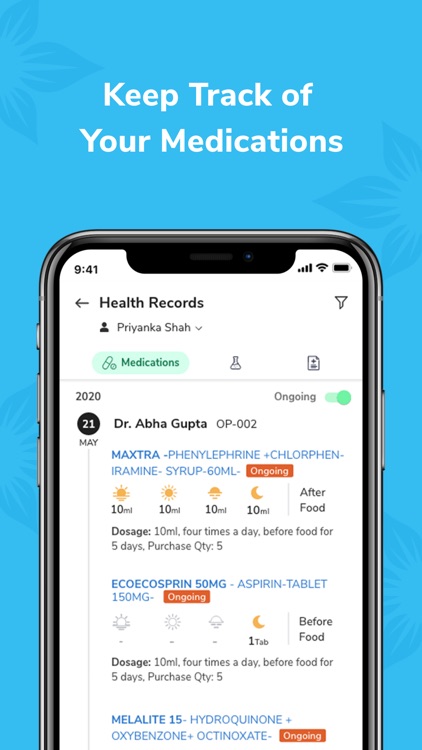The image showcases a mobile application interface designed to assist users in tracking their medications meticulously. The interface prominently features a title that reads, "Keep Track of Your Medications," and is organized under the health records of a user named Pyrankasai. 

The current view is focused on the "Medications" tab, highlighting the section where users can monitor their medication schedules. The displayed entry is dated May 21st, 2020, and is associated with Dr. Abha Gupta, identified by the code OP-002.

The medication list includes three entries, each with detailed dosages and instructions:
1. **Maxtra Syrup**: 60 milliliters - 10 milliliters four times a day before food, prescribed for five days. The purchase quantity indicated is five bottles.
2. **Echo Aspirin**: 50 milligrams - one tablet daily before food.
3. **Melolite 15**: Contains oxybenzone, octinoxate, and hydroquinone. No specific dosage or instruction details are provided for this medication.

Each medication entry is accompanied by icons and instructions representing the time of day and specific instructions such as "after food" and "before food". Status indicators show each medication entry with an "ongoing" red status label, suggesting that the patient is currently on these medications.

The app interface appears user-friendly, structured to ensure that users can easily manage and adhere to their prescribed medication regimens accurately and effectively.